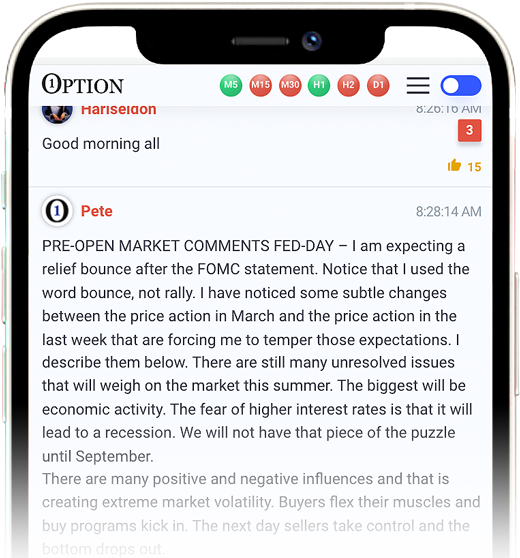In the image, a screenshot is displayed featuring what appears to be either an app interface or a blog post. At the top, the word "Option" is shown with the character "1" integrated into the "O," possibly indicating "Option One." Adjacent to this title are a series of circular buttons: a green button labeled "MS," a red button labeled "M15," another red button labeled "M30," a green button labeled "H1," a red button labeled "H2," and another red button labeled "D1."

Beneath these buttons, there are three horizontal lines arranged vertically, likely representing a menu icon. There is also a switch visible, although its specific function is not clear from the image.

Further down, a profile picture of a user named Haris Dian Mercedian is visible alongside his name. Below the profile, there's a message reading "Good morning all," followed by the "Option" title with the integrated "1" logo. The message pertains to "Pete" discussing pre-open market comments on "Fed Day," suggesting the content is related to business news, specifically about the Federal Reserve’s latest announcements on interest rates.

The post was made at 8:28 a.m. and has received 15 likes.